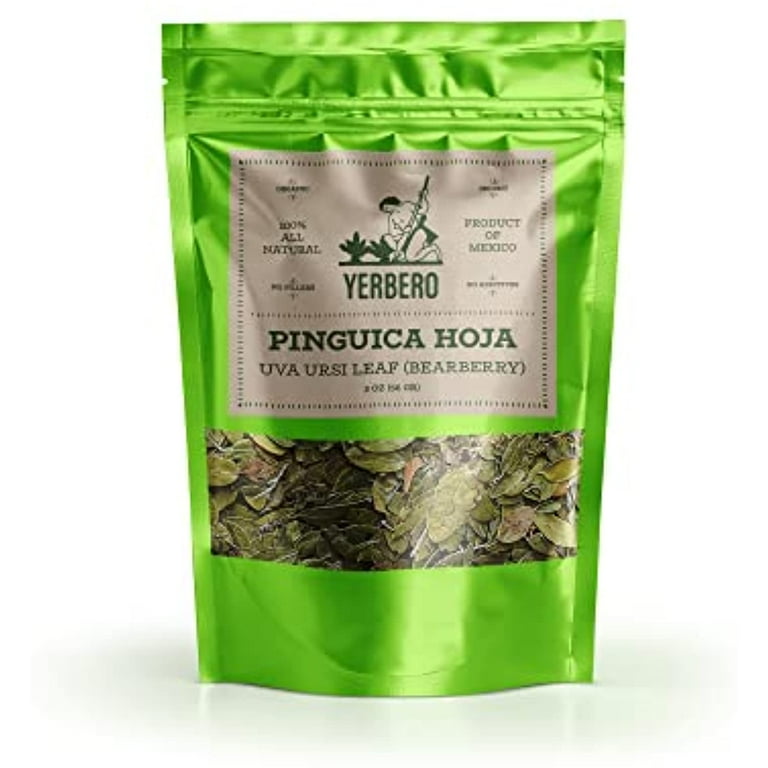This image features a resealable green foil aluminum bag containing eight ounces of dried herbs. The packaging is a vibrant lemon or neon color at the back, and it has a clear transparent section at the bottom where the crushed, dried herb leaves can be seen. The product is categorized as Bearberry or Uva (Sea Leaf) with the botanical name "Pinguica Hoja." The front label prominently displays "Yerbero," the brand name, in green font against a brown background.

Central to the label is an illustration of a person kneeling on a farm, engaged in harvesting plants with a tool, conveying a commitment to natural farming practices. The label also emphasizes that the herbs are "100% All Natural." On the right side, the label states that this is a "Product of Mexico."